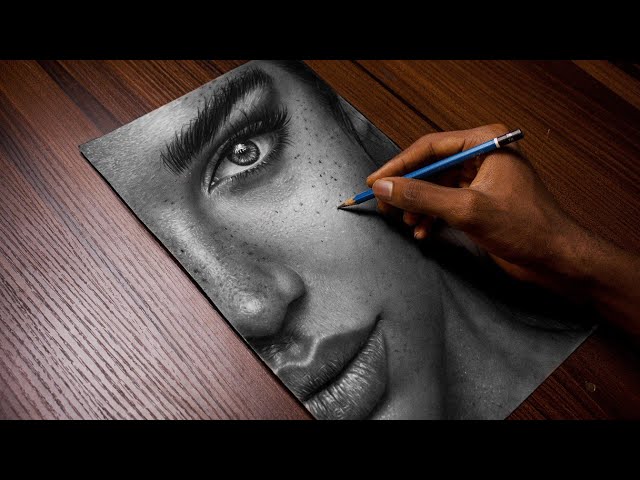The image depicts a detailed, photorealistic scene of a dark-skinned hand holding a blue pencil, actively sketching a close-up portrait of a woman on a dark oak table. The woman's face, drawn in pencil, shows only one eye, most of her nose, and half of her lips and jaw, with her eye staring directly at the viewer. She has full lips, various freckles—particularly on her cheeks and nose—dark, bushy eyebrows, and dark hair. The right side of the image is visibly darker than the left, where the table reflects light, enhancing the photograph's realistic quality.